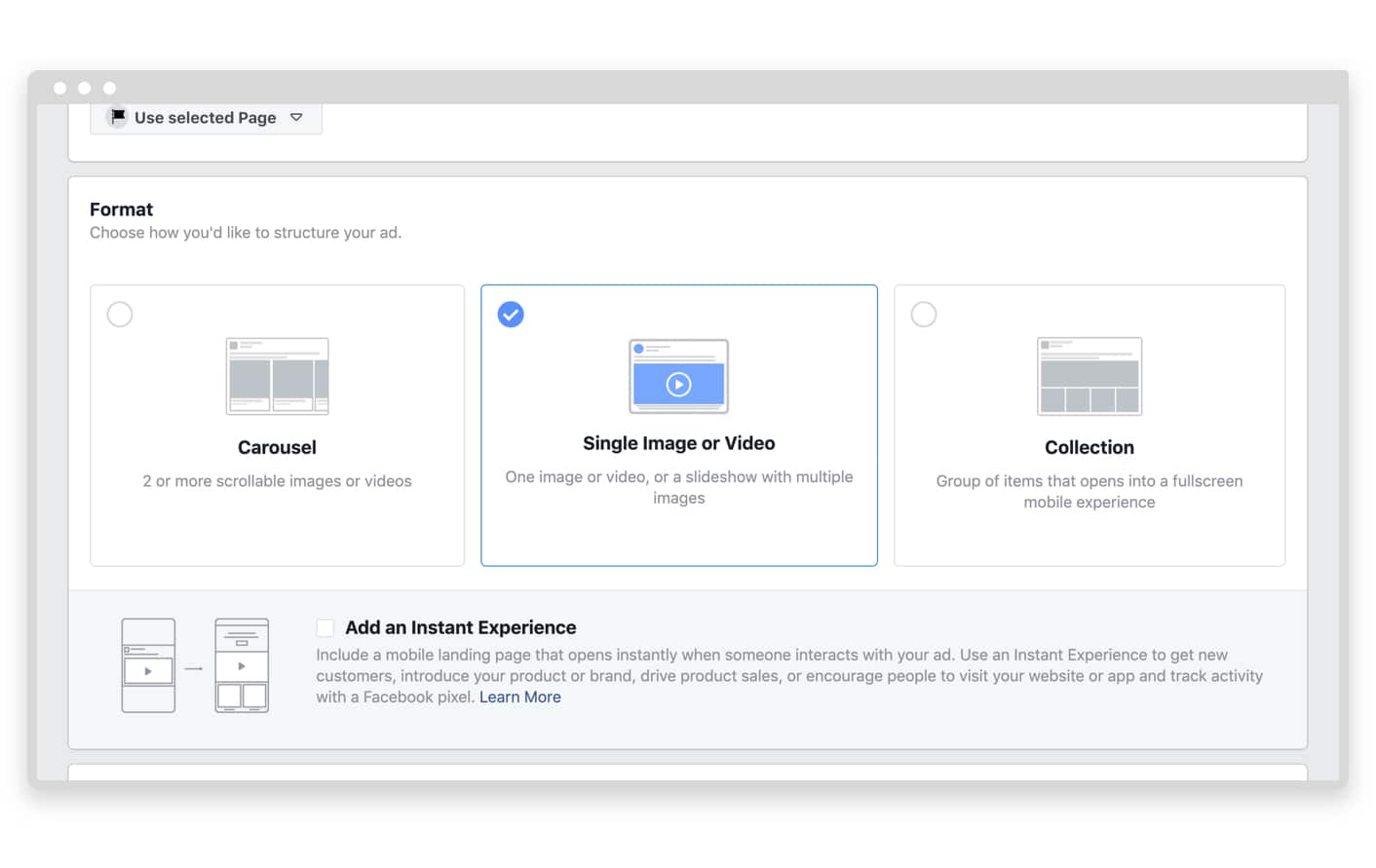The image depicts an upload page on a website accessed through a Mac browser, identifiable by the iconic three circular control buttons in the top left corner of the window, each colored white. The background of the page features a patterned design, blending grey hues with white squares.

In the top left corner, a dropdown button labeled "Use Selected Page" is visible, accompanied by a black flag icon to its left. Dominating the center of the page is a white interface box. This box prominently displays "Format" in the top left corner, with a description underneath that reads, "Choose how you would like to structure your ad."

Below this description are three selectable tabs: 
1. "Carousel" - for two or more scrollable images or videos.
2. "Single Image or Video" - which is currently marked as selected.
3. "Collection" - described as a group of items that opens into a full-screen mobile experience.

At the very bottom, there's a light grey horizontal bar that provides an option to "Add an Instant Experience," accompanied by a checkbox that can be selected to enable this feature.